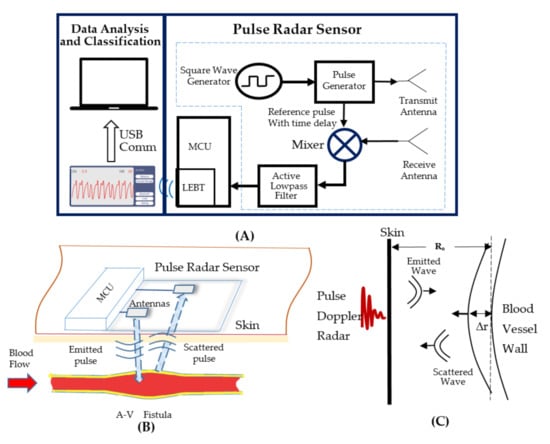This image is a detailed chart illustrating the components and functionality of an alphagraphic data analysis and classification pulse radar sensor system. At the top, the chart is divided into two sections. The left section, labeled "Data Analysis and Classification," features a graphic of a laptop with an arrow labeled "USB-COMM" pointing toward it, indicating the communication interface. Below the laptop, there’s a squiggled red line representing data visualization.

The right section of the chart, labeled "Pulse Radar Sensor," contains a comprehensive flowchart starting with a "Square Wave Generator" followed by various components such as ovals and rectangles labeled "Pulse Generator," "Transmit Antenna," "MCU" with "LEBT," and "Active Low Pass Filter." The flowchart includes lines and arrows illustrating the connection and flow of the radar pulse, with a Y-shaped line symbolizing the "Transmit Antenna" and another pathway involving a "Mixer" and "Reference Pulse with Time Delay."

At the bottom of the image, there is a close-up diagram in color marked "Pulse Radar Sensor," showing the device from a different perspective, likely highlighting its physical constituents. To the right, the chart ends with a graph labeled "Pulse Doppler Radar," which visually represents the radar's capability to detect anomalies in blood vessels and how the collected data is analyzed and displayed on a computer.